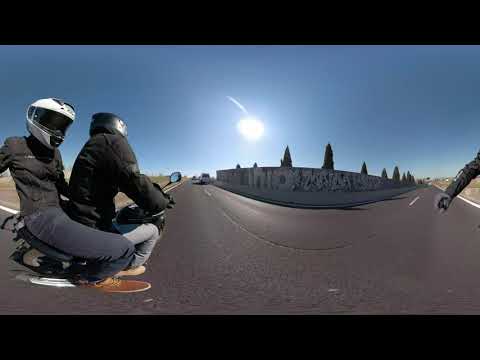The photograph captures a dynamic selfie of two motorcyclists riding a small black motorcycle on a dark asphalt road marked with a dotted white lane divider. The motorcycle driver, dressed in a black padded jacket, dark gray pants, and brown shoes, wears a black semi-glossy helmet and appears to be looking away from the camera. The passenger, holding onto the driver's waist, sports a white helmet, a black jacket, black denim jeans, and light brown shoes with white bottoms. The backdrop features a clear blue sky with the sun depicted as a bright circular white light. A curious detail is the oblong lens effect, slightly warping the nearest objects. In the right part of the image, a low white wall covered in colorful graffiti runs parallel to the road, with green conical trees peeking out from behind it. Additionally, a random hand and arm are visible on the right side, adding a sense of spontaneity to the composition.